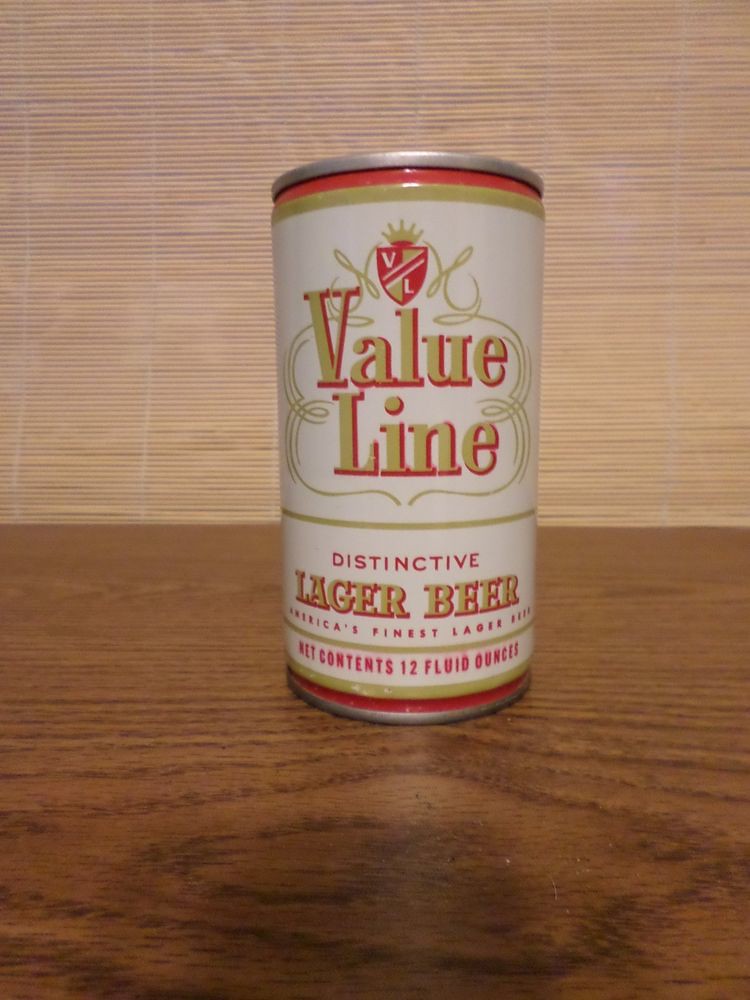In this close-up vertical photograph, a can of beer is prominently featured standing upright on a medium-dark brown, wood-grain table with notable knots and darker streaks. The background showcases tan and light brown blinds that are pulled down, occupying the upper half of the image, while the table covers the lower half. The beer can itself has a distinctive design. The top and bottom parts are silver, and the main body of the can is predominantly white. 

In the middle of the can, the brand name "Value Line" is displayed in gold letters with a red outline. Above this text, there's a red, white, and gold crest featuring a golden crown atop. In the crest, the left corner holds a white "V" on a red background, and the right bottom corner holds a white "L." A horizontal golden line runs across the can, separating various text elements.

The words "Distinctive" in red and "Lager Beer" in gold are prominently displayed below the crest, with "America's Finest Lager Beer" in smaller red letters underneath. At the bottom of the text, it mentions "Net Contents 12 Fluid Ounces" in red. There is also intricate embroidery around the words "Value Line," adding a decorative touch to the can's design.